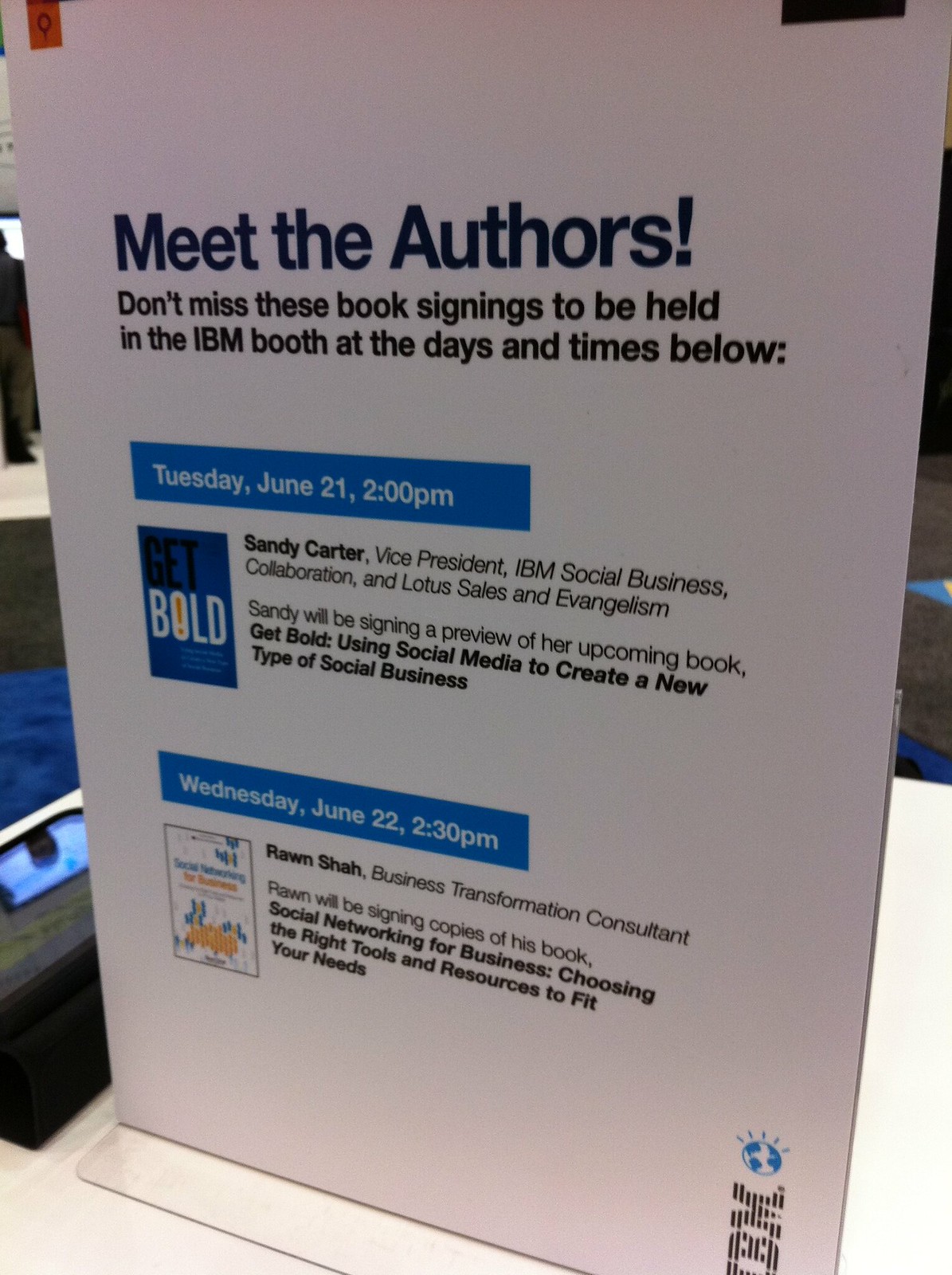In the image, there's a cardboard billboard standing on a white table with a white backdrop, promoting author signings. At the very top, in bold black letters, it reads "Meet the Authors!" Beneath this, in smaller black letters, it states, "Don't miss these book signings to be held in the IBM booth at the times and dates below."

Below this heading, against a blue background, the first event is highlighted: "Tuesday, June 21st, 2 PM," featuring Sandy Carter, Vice President of IBM Social Business Collaboration and Lotus Sales and Evangelism. Sandy will be signing a preview of her book, "Get Bold: Using Social Media to Create a New Type of Social Business." Accompanying this information is a picture of the book cover which simply reads, "Get Bold."

Following this, the second event is listed: "Wednesday, June 22nd, 2:30 PM," where Ron Shah, a Business Transformation Consultant, will be signing copies of his book, "Social Networking for Business: Choosing the Right Tools and Resources to Fit Your Needs." A picture of Ron's book cover appears next to this text.

In the bottom right corner of the billboard, the IBM logo is displayed. The background of the setting includes some glimpses of blue and brown.